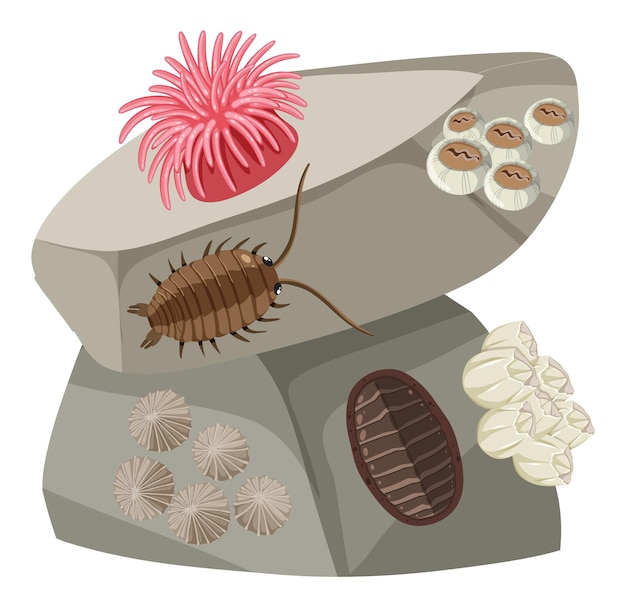The illustration depicts a detailed underwater ecosystem resembling an ancient coral reef, set against a white background. Central to the image are two large stones stacked vertically. The top stone, flat and colored in shades of gray and tan, supports a vibrant, coral pink sea anemone with numerous spongy protrusions. Five barnacles cling to its right side, and a brown isopod with dark brown central markings, black eyes, and long antennae crawls across its surface. The bottom stone, resembling a more rounded rock, also features multiple barnacles on its right side and scallop shells attached to its left. A second isopod is partially visible from the underside of this stone. Other small, cream-colored objects punctuate the scene, adding to the rich tapestry of this animated yet ancient seascape.